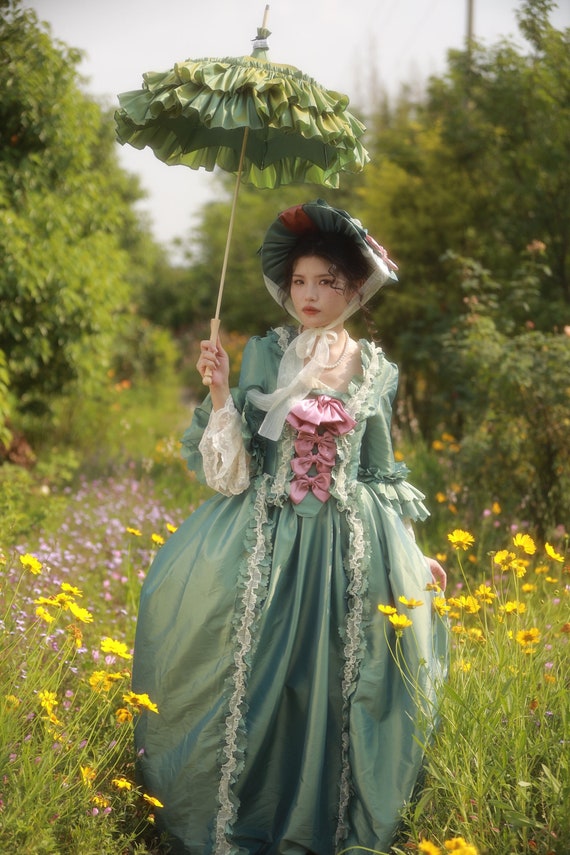In the image, an Asian lady is standing gracefully in a picturesque field of wildflowers, dressed in attire reminiscent of the Victorian era. She wears an elegant long, flowing sage green satin dress adorned with two rows of lace trim cascading from her shoulders to the hem. Her dress has poofy sleeves with cream-colored lace extending down to her wrists, and four pink bows arranged across the center of her chest and stomach. Tying her ensemble together, she dons a large green bonnet secured with a cream-colored ribbon under her chin and accessorizes with a pearl necklace. In her right hand, she holds a multi-tiered ruffled green parasol made of a luxurious material such as silk or satin. The backdrop features a densely wooded area with tall trees, high grass, and vibrant wildflowers in shades of yellow and purple, set against a gray, cloud-covered sky. The overall setting appears to be a lush orchard, highlighting the serene beauty of a spring day.